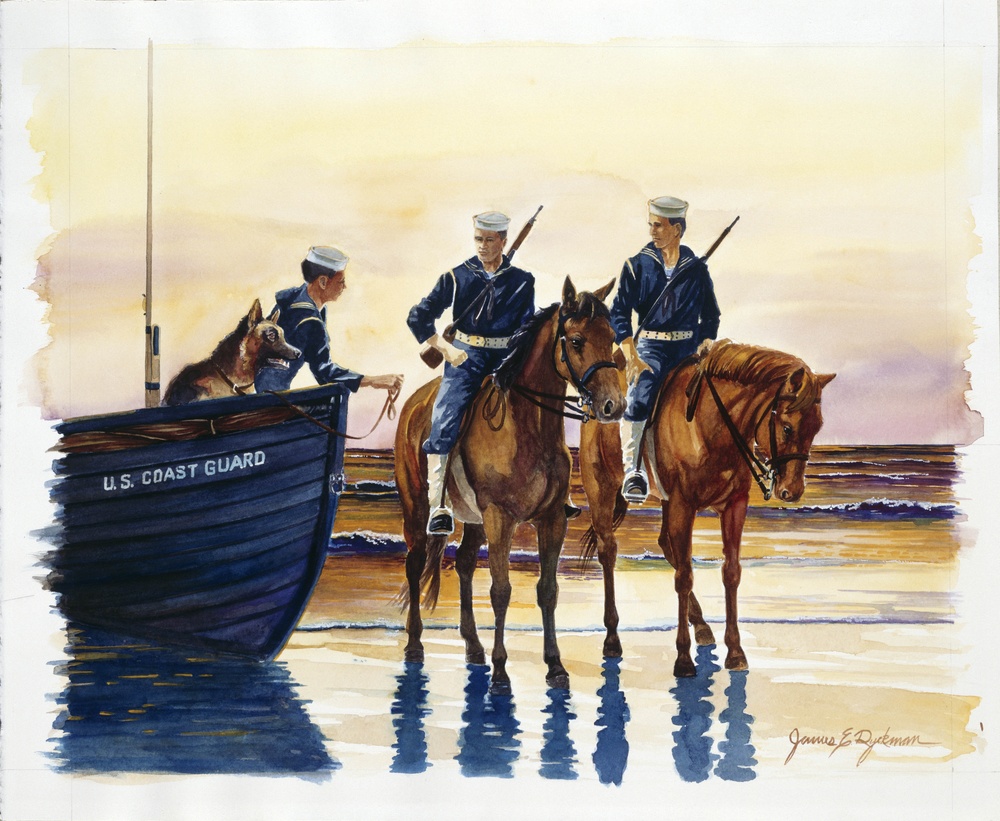This detailed painting depicts a scene involving the U.S. Coast Guard. Set on a beach near calm, reflective waters with small waves, the artwork is imbued with a palette of dark navy blues, yellows, pinks, and purples. The sky's warm hues create a striking backdrop for the action on the shore. In the foreground, two Coast Guard soldiers, dressed in blue uniforms with white belts, shin coverings, boots, and traditional white navy hats, sit atop large brown horses. They have rifles strapped to their backs. Nearby, a smaller wooden U.S. Coast Guard boat, partially visible and painted navy blue with white text, is stationed on the left. A third soldier in the same uniform stands aboard the boat, alongside a brown and black German Shepherd, extending a rope to the men on horseback. The wet sand of the beach reflects these figures vividly. The artist’s signature can be found in the bottom right corner of this evocative watercolor painting, adding a touch of authenticity to the historical scene it portrays.